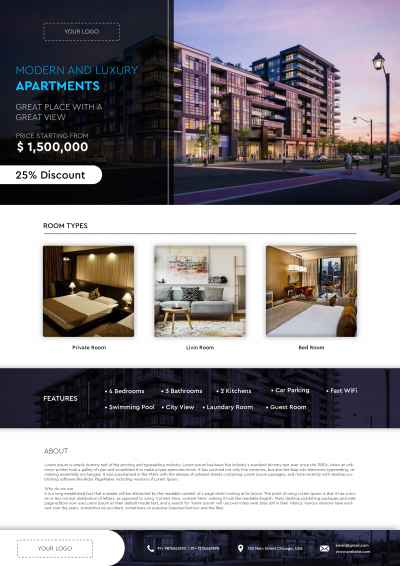On the website showcasing modern and luxury apartments, the top section features a prominent black box on the left-hand side, containing details about the apartments. The text highlights the luxurious nature of the apartments, boasting an exceptional view and mentioning that prices start from $1.5 million after a 25% discount. Adjacent to this black box, on the right, is a captivating image of the modern and luxurious apartment building itself.

Beneath this top section, the website provides a detailed overview of the various room types available. There are three options listed: private rooms and two other room types (one of which is unreadable from the capture). Directly below this section, a wide black box spans the page, listing the numerous features of the apartments, including four bedrooms, three bathrooms, two kitchens, car parking facilities, a swimming pool, and more.

The following section features an "About" box that provides a thorough history and description of the apartments, outlining the goals and scope of the project. At the bottom of the webpage, there are options for co-branding. There are spaces allocated for your logo both at the top of this section and at the bottom, along with fields for contact information.

Overall, the webpage appears to be a comprehensive template designed to be customized and implemented by real estate businesses focused on selling modern and luxury apartments.